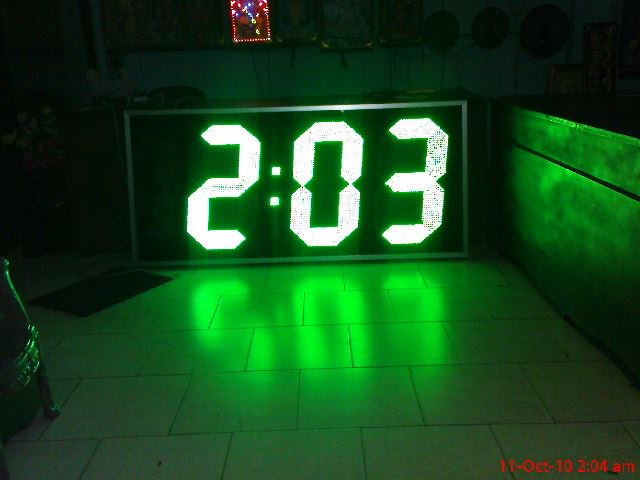This photograph captures a striking scene of a large digital clock glowing in the darkness. The clock, likely resembling one removed from a scoreboard, dominates the image with its vivid green digits displaying the time as 2:03. The reflective properties of the white tile floor create an intriguing visual effect, transforming the green numbers into an illusion of 5:07. The room itself is enveloped in a moody ambiance, the glow from the clock casting a faint luminescence on the surrounding walls. In the background, a square section of the wall is illuminated with a vibrant mix of red, blue, and white lights, adding depth to the scene. A small red watermark at the bottom right corner of the photograph records the date and time of capture as 11-October-10, 2:04 a.m., contributing to the overall mystique of this nocturnal image.